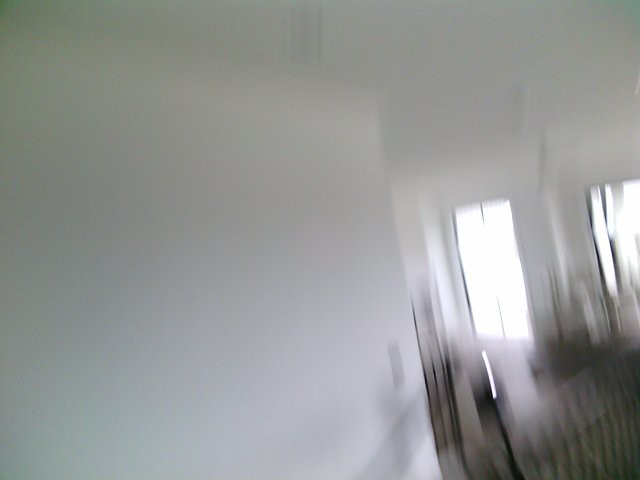The photograph captures an interior scene from a high vantage point, slightly angled downwards. Although the image is somewhat blurry and out of focus, various elements of the room are distinguishable. On the left side of the frame, a white, slanted wall runs across approximately two-thirds of the image, adorned with gray shadowing near its base. In the background, additional white walls and a white ceiling can be seen. The far end of the room features a bright glass door which floods the space with light. Flanking the door are windows dressed with white curtains. The floor is a warm brown hue, and the lower right corner of the photo includes indistinct black lines, the details of which are not clear.